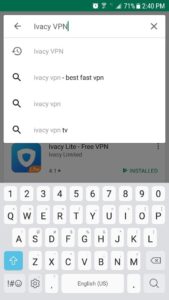The image features a smartphone interface against a light gray background. At the top of the screen is a status bar displaying "2:40 PM" and a battery level of "71%". Below the status bar is a green notification box displaying the same time and battery information. 

Centered on the screen is a white pop-up window titled "IVACY VPN", with a left-pointing arrow on the left edge, an "X" button on the right, and a small clock icon with a circular arrow next to "IVACY VPN". Beneath this, a search bar displays various suggestions: "IVACY VPN", "Best Fast VPN", "IVACY VPN TV".

The bottom section shifts to a gray background with a blue box featuring a white triangle and yellow accents at the bottom, labeled "IVACY Life Free VPN". There's a right-pointing arrow next to an "Install" button. 

The on-screen keyboard is also shown, featuring white keys with black letters on a light gray background. On the left, a blue key has an upward-pointing arrow, adjacent to a utility key with symbols like exclamation points and hashtags. There's also a button with a settings cog, a key for switching languages, and a punctuation key. On the right side, a magnifying glass button for search is placed below a key marked with a square "X" icon.